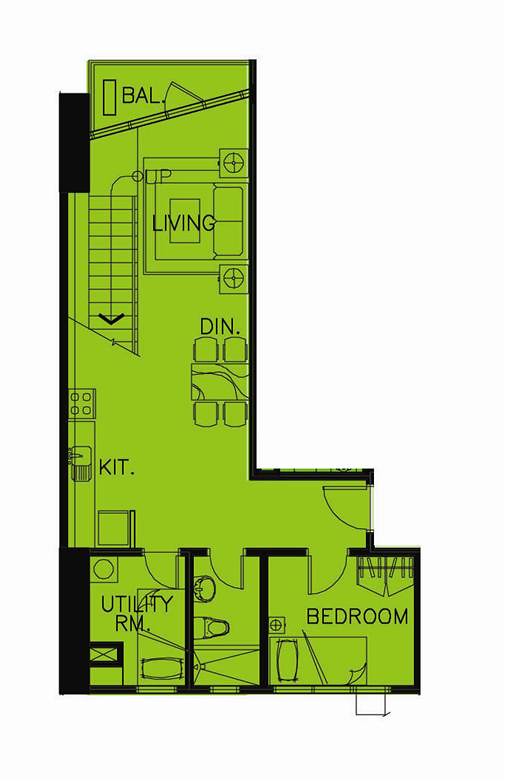This architectural drawing depicts a one-bedroom apartment plan, outlined in black with the apartment area highlighted in green. At the top of the layout, a spacious balcony is visible, providing outdoor space for residents. Upon entering the apartment, there is a staircase leading to or from an upper level, suggesting a multi-level design. Adjacent to the stairs is a living area, furnished with a couch and a pair of side tables, creating a cozy space for relaxation.

Further into the apartment, a dining area with a table and four chairs is situated across from the kitchen, allowing for easy access and convenience during meal times. The kitchen features essential appliances and cabinetry arranged below the staircase area, optimizing the apartment's spatial design.

Towards the bottom of the drawing, three specific rooms are shown: the utility room, the bathroom, and the bedroom. The utility room appears to have water connections, possibly indicating the presence of a sink or laundry facilities. The bathroom includes fixtures such as a sink, a toilet, and a shower, designed for complete functionality. Lastly, the bedroom contains a bed, a dresser, and a closet area, providing ample storage and comfort for residents.